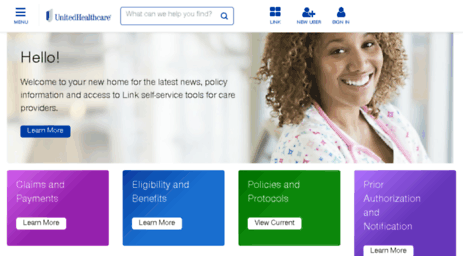A screenshot from the UnitedHealthcare website showcases a well-structured layout with multiple elements. At the very top, a horizontal navigation bar spans across the screen, prominently featuring the UnitedHealthcare logo in the top left corner, rendered in blue. Adjacent to the logo is a white search bar outlined in blue, containing the placeholder text "What can we help you find" and a blue magnifying glass icon on its right side. 

To the right of the search bar, three blue buttons are aligned horizontally. Below this navigation bar, a prominent banner stretches across the width of the page, displaying the image of a smiling healthcare worker with light brown skin and curly brown hair. 

On the left side of the banner, a welcoming message reads: "Hello, welcome to your new home for the latest news, policy information, and access to link, self-service tools for care providers." Directly under this text is a blue button labeled "Learn more."

Further down the page, four columns with different colored squares are arranged, each presumably representing various sections or features available on the site.